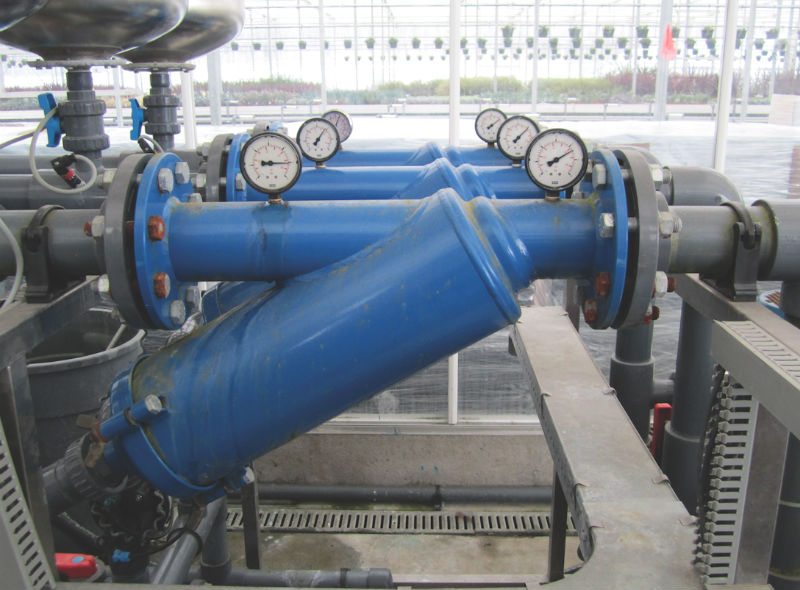The image showcases a complex piping system, likely part of a water treatment or hydroponics farm, potentially within a greenhouse. Central to the setup are blue metal cartridges approximately 2 feet long, each flanked by 8-volt flanges made of gray PVC piping, about 2 inches in diameter. Along these pipes, there's a noticeable array of pressure gauges, strategically placed at both ends of the blue cartridges, their needles pointing to different readings. One key component includes a backflow valve topped with a black pressure tank or bowl. Below the flanges, several gray rubber trash cans are positioned, with red shutoff valves visible on the ground. The infrastructure features drainage grates for water management. In the backdrop, the space opens to a greenhouse environment with multiple tiers of plant shelving, nurturing various plants, emphasizing the role of the irrigation system in supporting the facility's agricultural activities. The scene includes elements of concrete, metal, and stone, creating a stark industrial aesthetic interspersed with the vibrant blue of the pipes, indicating their likely importance.